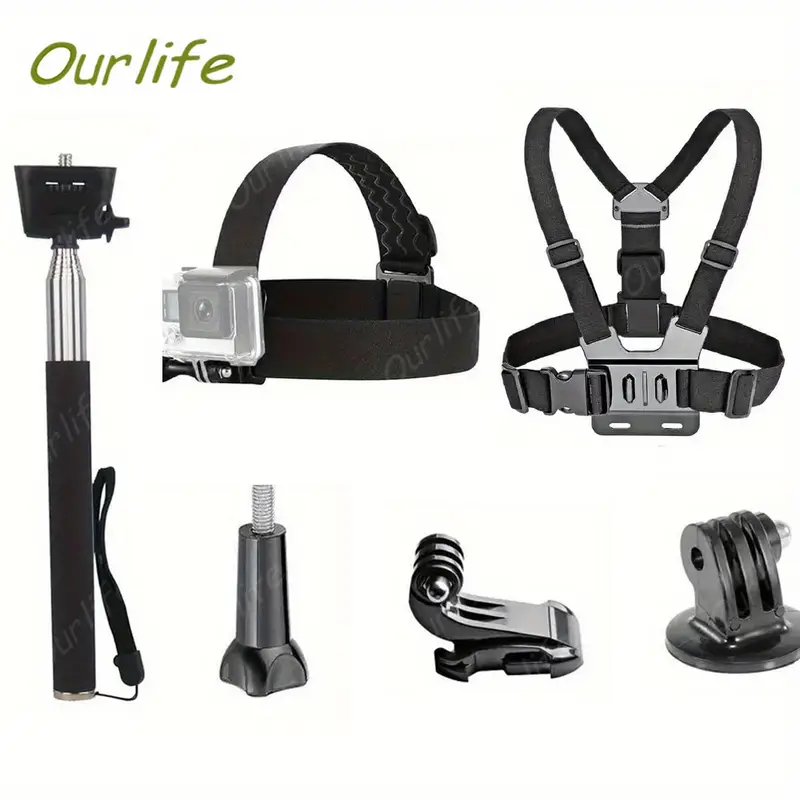The photograph is a detailed promotional product image showcasing various black and gray accessories for a GoPro camera. On the left side, there's an expandable monopod, typically used as a selfie stick, featuring a clamp at the top for securing the camera. Beside it, there's a head strap designed for mounting the camera on a helmet or directly on the forehead, providing a first-person perspective. Moving right, there is a body harness with suspenders that clip around the shoulders and waist, meant for hands-free filming. At the bottom of the image, there are three smaller accessories: a screw-in mount adapter, and two curved mounts that can be adjusted to change the height and angle of the camera. The overall layout is organized, highlighting the versatility of the mounting options for action filming. The image also includes a sign that reads "Our Life" in green letters, with a capital "O" and lower-case letters for the rest, adding a personal touch to the promotional setup.